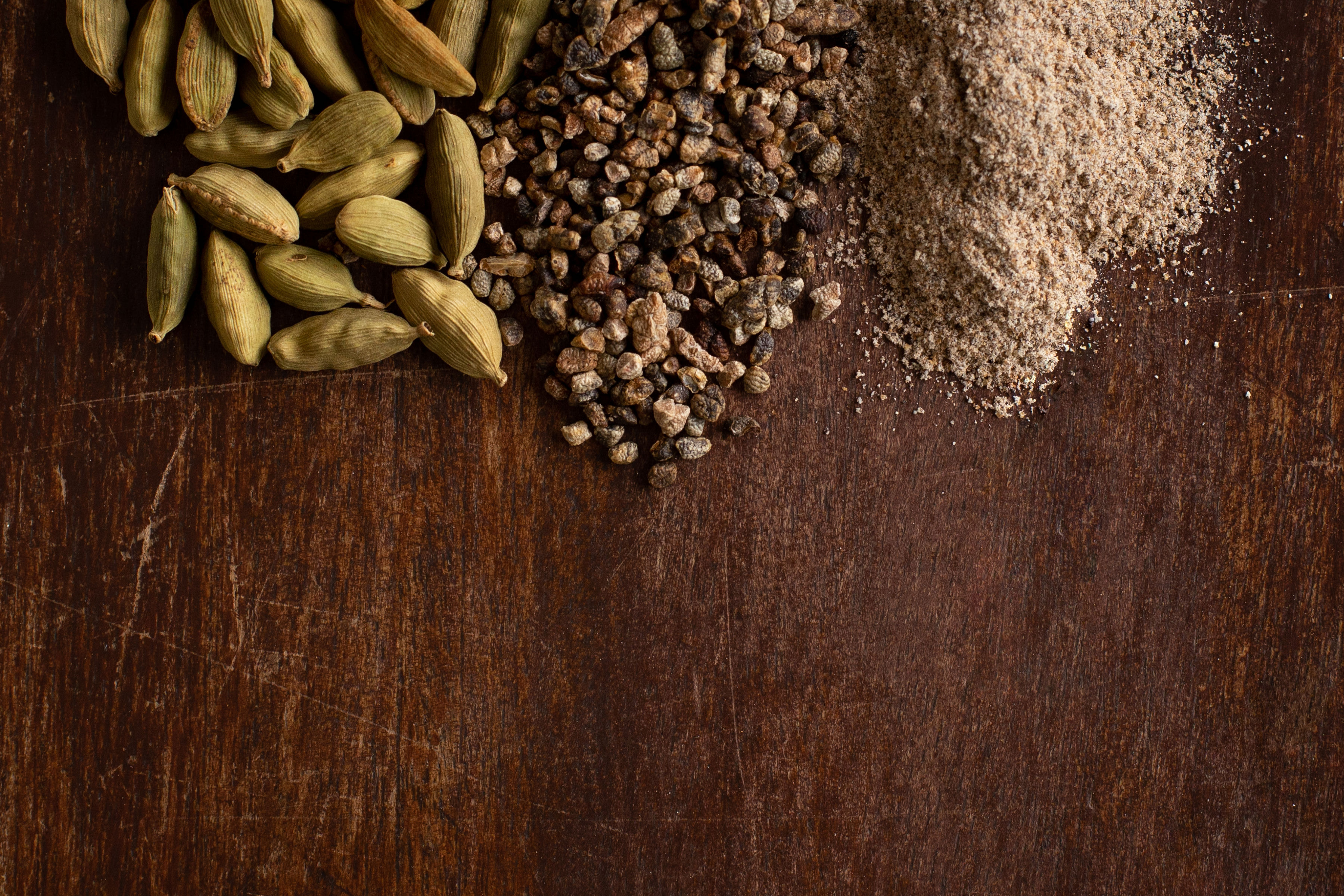This overhead close-up image features three distinct piles of seeds in different stages of grinding, arranged on a dark, scratched wooden surface that might be a table or a cutting board. The left pile consists of roughly 30 light yellow pods, resembling peanut-sized dried seeds with a texture similar to a corn husk. In the middle, the seeds are revealed and appear as variously colored small chunks, showcasing hues of brown, tan, white, and gray. The rightmost pile is a fine tan dust, indicating the seeds have been ground down to a powdery consistency.